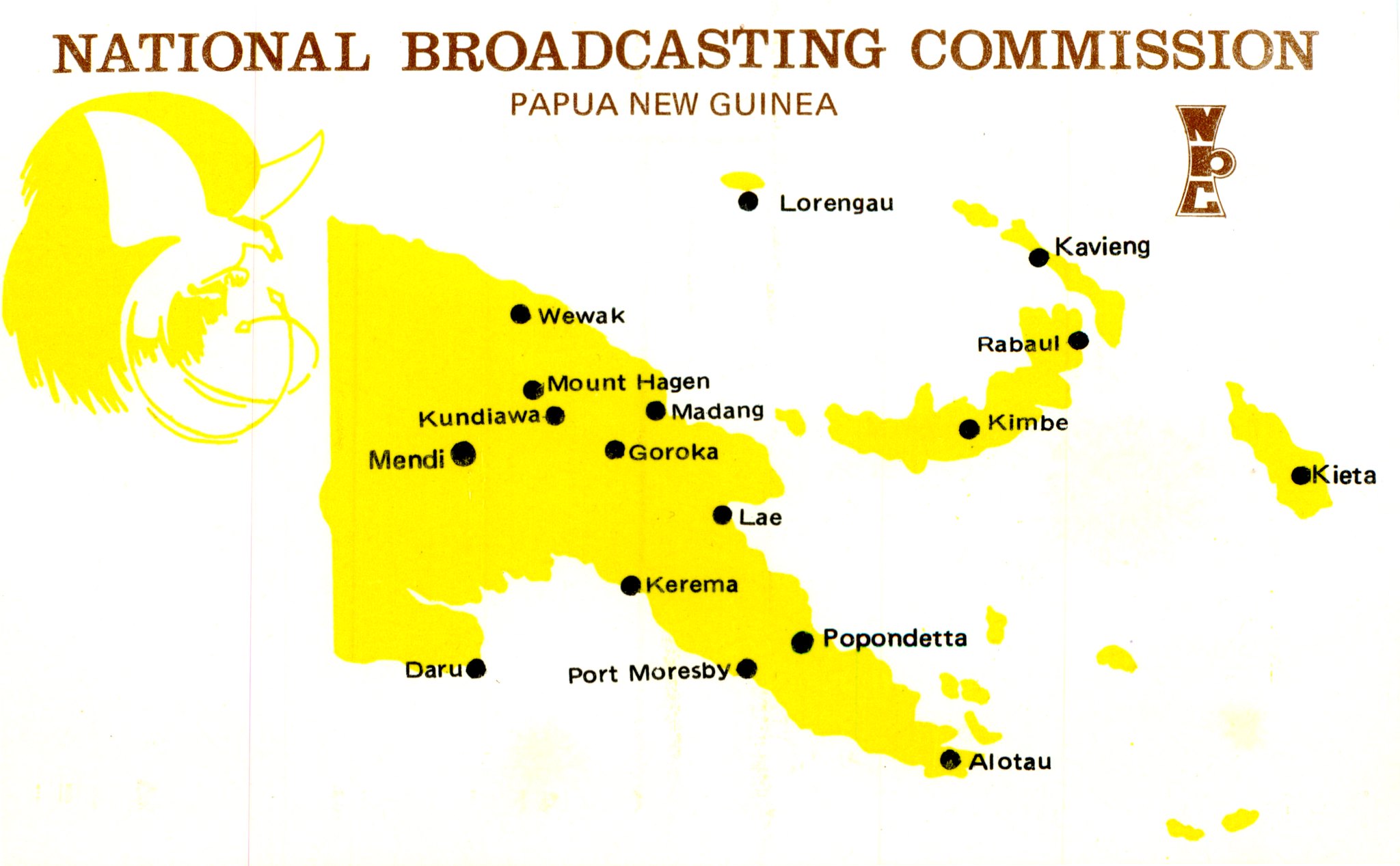The image is a detailed map of Papua New Guinea on a white background. The very top of the image features the words "National Broadcasting Commission" in large, brown, uppercase letters. Directly below, in smaller uppercase letters and also in brown, it reads "Papua New Guinea." On the left side of the map is an illustrated logo of a bird, likely a bird of paradise, depicted in yellow against the white backdrop. The bird has a graceful, long tail and is oriented so that it appears to be looking towards the map. The central focus of the image is the map itself, showing the landmasses of Papua New Guinea in yellow. Major cities across the islands are marked with black dots and their names are listed in black text. Notable cities such as Port Moresby, Daru, and Olato are among approximately 20 cities identified on the map, providing a clear geographical representation of the nation.